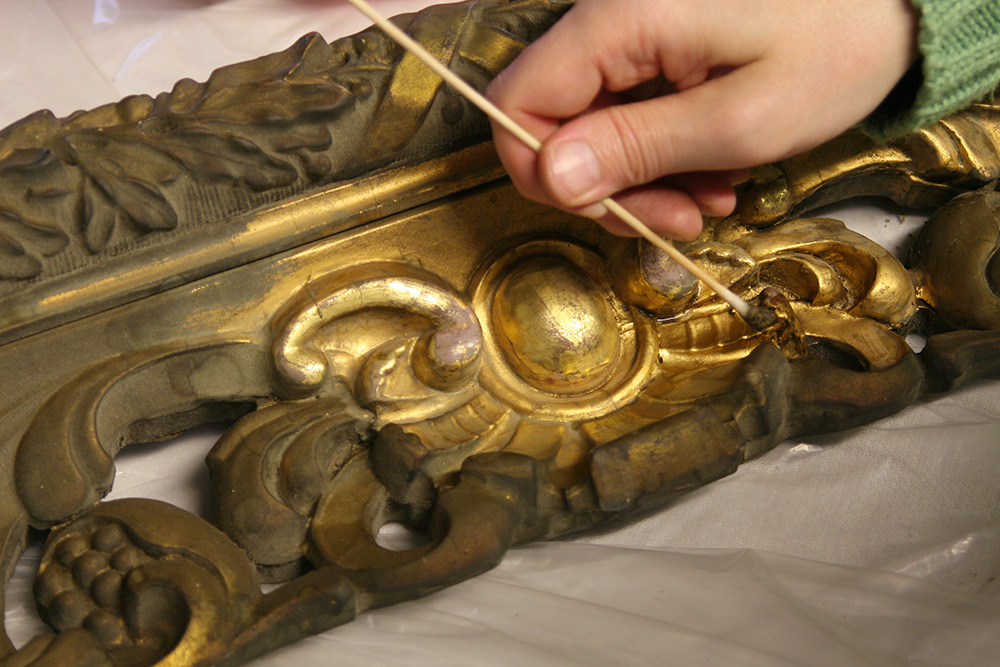The photograph showcases an intricately designed, ornate gold frame with a bronze tint, adorned with floral etchings and engravings. The frame, which appears shiny and clean in the center but dull around the edges, lies on a lavender-colored plastic sheet. A hand, wearing a green sweater sleeve, extends from the top right corner, holding a long cotton swab, visibly dirty at the tip, indicating active cleaning. The person's meticulous effort to clean out the frame's crevices is gradually restoring its bright, gold sheen, especially evident in the intricate flowery patterns and the central bronze emblem.